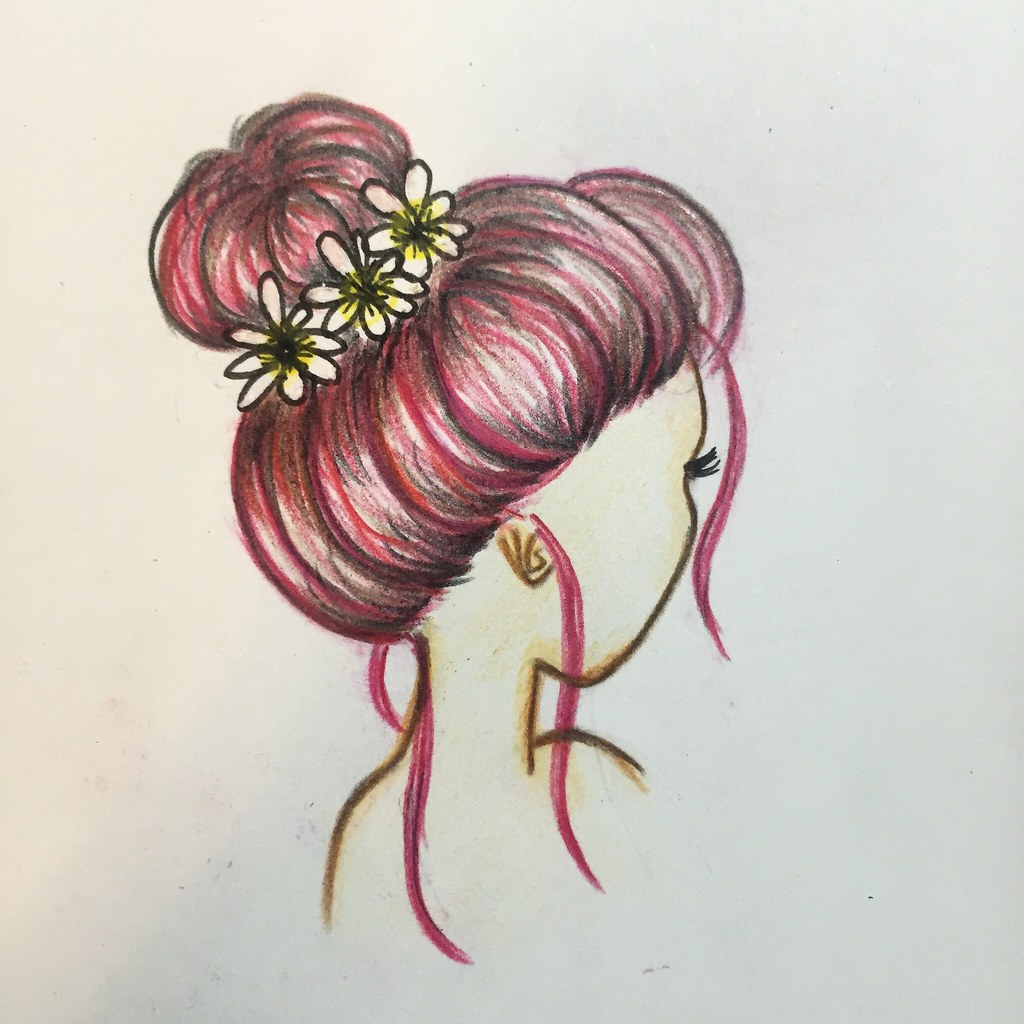This is an image of a detailed, hand-drawn artwork on white paper. The subject is a woman viewed from her shoulders up, looking away so only the side of her face is visible along with her long black eyelashes that accentuate her one visible eye. Her hair, rendered in various shades of red and brown, is styled in a top knot bun. Surrounding the bun are three white flowers, which resemble daisies with yellow and black centers. Several strands of her bright red hair hang down, two framing her face at the front and two others trailing at the back of her neck. Additionally, a possible gold earring is noticeable near her ear. The overall drawing appears to be done in colored pencils or crayons, with the background remaining plain white, making the central figure in the artwork stand out vividly.